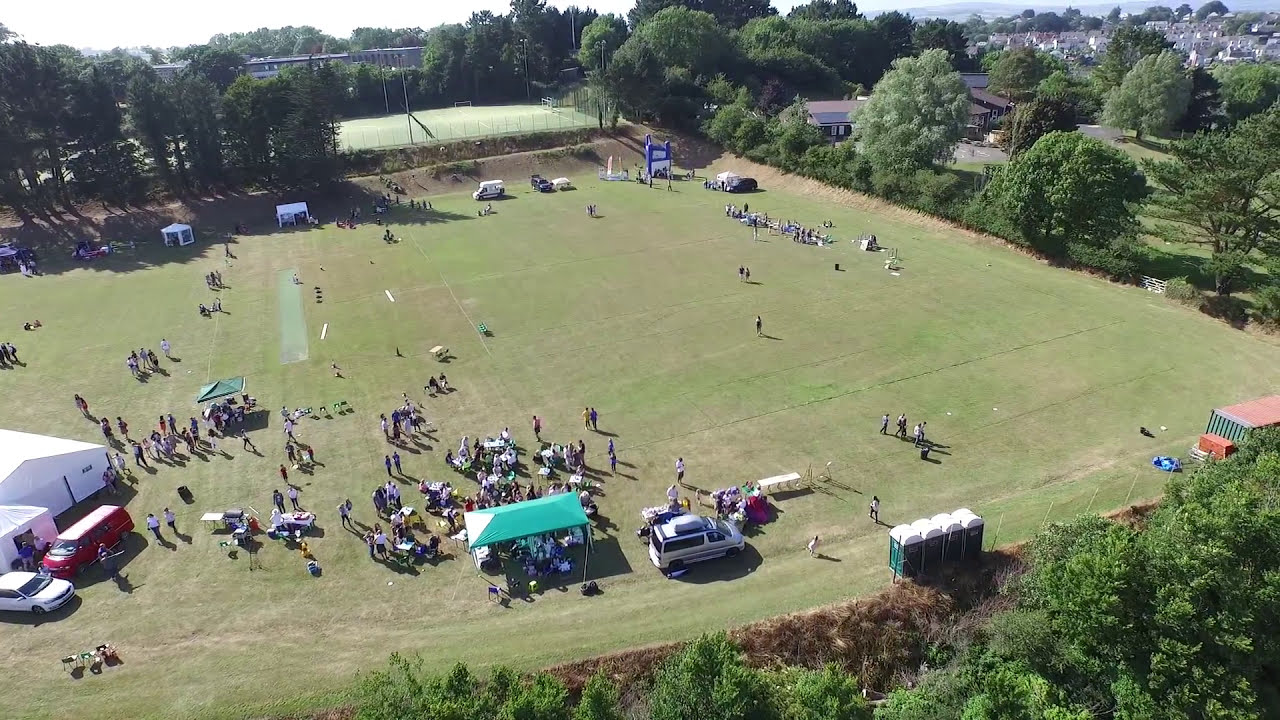This color photograph, captured from a bird's-eye view using a drone, showcases an extensive grassy playing field occupying most of the image. The grass is freshly mowed, with some patches appearing slightly barren and brown. Scattered throughout the field are numerous people, resembling tiny ants due to the aerial perspective. Toward the bottom left quadrant, a prominent blue pop-up tent is visible, surrounded by groups of people. Adjacent to this tent are several vehicles and a white-tinted temporary structure. In the bottom right corner, a row of approximately four portable toilets is lined up near more parked cars. The field is encircled by large green trees, creating a natural border. In the background, particularly in the top right section, clusters of buildings are interspersed among additional tree coverage. The scene is set outdoors in the middle of the day, bathed in natural light, and gives off a sense of realistic, representational photographic style. The colors evident in the scene include varying shades of green, brown, orange, gray, tan, red, and turquoise.